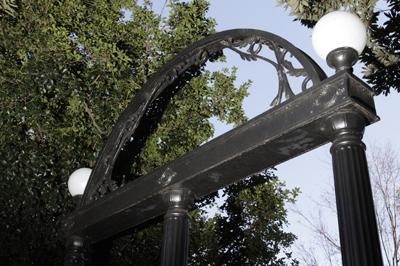In this photograph, taken from an eye-level perspective looking slightly upwards, we see an ornate black metal archway structure set in an outdoor park. The archway comprises three vertical black columns embellished with vertical lines, connected by a horizontal beam that spans from the first to the third column. Above the columns, the beam extends into half-circle metal designs with intricate filigree patterns mimicking trees and leaves. Atop the first and third columns sit round streetlights. The scene is captured during the daytime under a clear sky, with verdant foliage framing the image; on the left side, leaves dominate from the top almost entirely to the middle, while on the right, a mix of blue sky and additional leaves can be observed in the top corner. The bottom portion of the structure is not visible, contributing to the focus on the detailed metalwork and the serene natural backdrop.